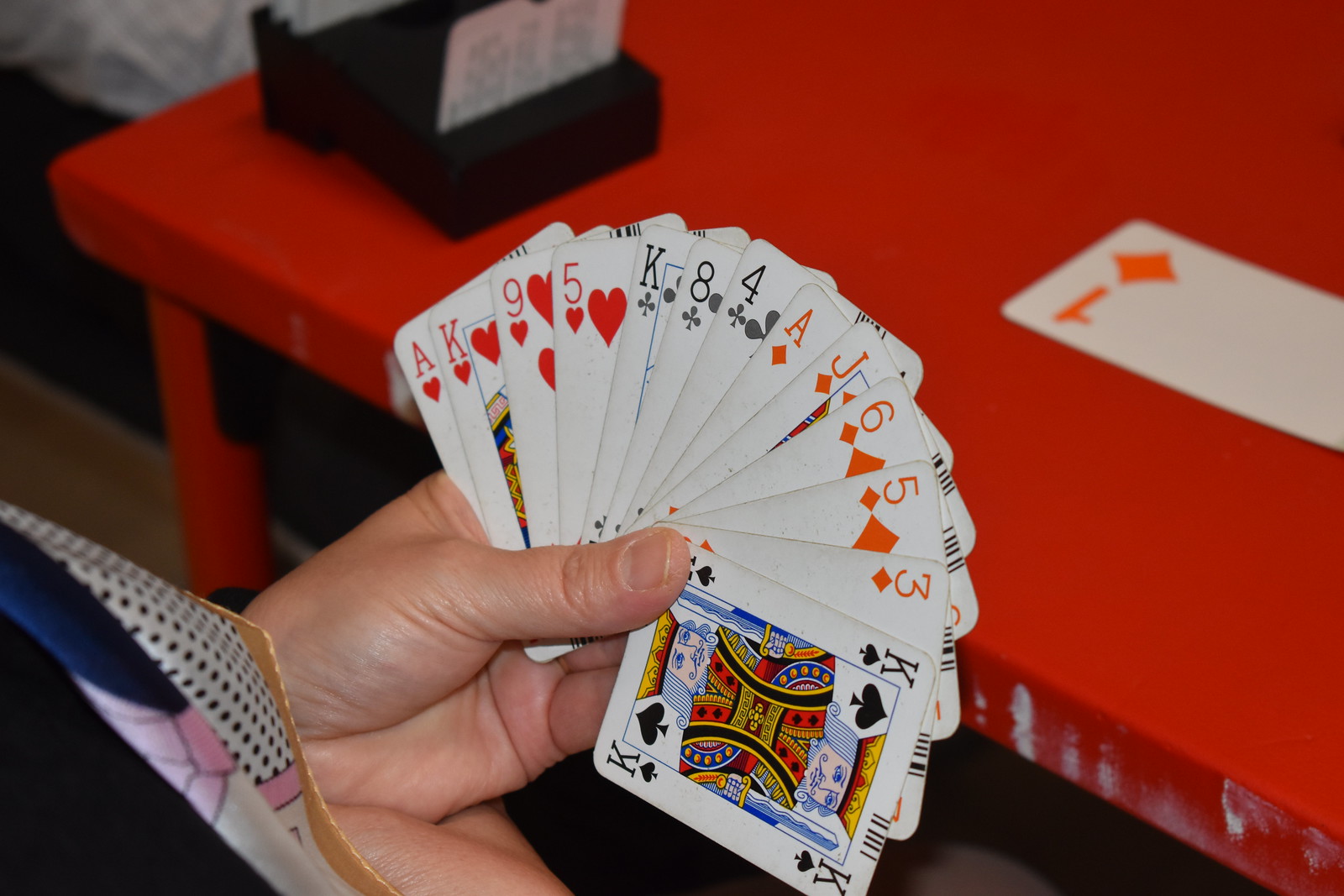An over-the-shoulder POV image captures an intense moment in a card game. A player's left hand holds a perfectly fanned-out set of thirteen cards, ranging from an Ace of Hearts to a King of Spades. The cards include an Ace of Hearts, a King of Hearts, a Nine of Hearts, a Five of Hearts, a King of Clubs, an Eight of Clubs, a Four of Clubs, an Ace of Diamonds, a Jack of Diamonds, a Six of Diamonds, a Five of Diamonds, a Three of Diamonds, and a King of Spades. The cards are held securely between the player's thumb and fingers, with the thumb pressing against the bottom left corners for support. Meanwhile, the right hand clasps gently around the left wrist, steadying the grip. The bright red table in front of the player contrasts with a single rectangular white card displaying the number "1" and a diamond symbol in orange lying flat on the table's surface. The angle of the shot, taken slightly from over the player’s right shoulder, provides a well-lit, immersive view of this strategic game moment.